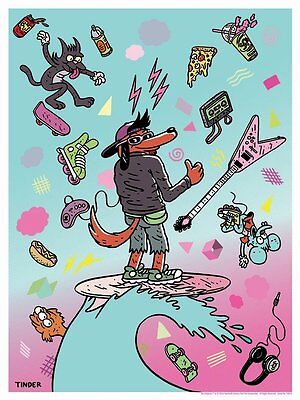The image features a vibrant cartoon illustration centered around a cool-looking dog character. The dog, drawn in a cartoon style reminiscent of animated TV shows from the '90s like "The Simpsons," stands upright on a surfboard, which is pink in the front and white in the back. The surfboard is riding a turquoise wave that comes up from the bottom of the image and curves to the right.

The dog has a brown fur coat, wavy black hair, and is sporting a backwards purple cap. He's wearing dark sunglasses, a gray jacket, and cutoff shorts with ragged edges. His feet, clad in green and white sneakers, are pointed to the right, and he is giving a thumbs-up with his right hand while his head is turned towards the viewer. He has a long nose and a red or brown tail that curves up to the left.

Surrounding the central figure are numerous colorful and whimsical elements. To the right of the dog is a pink, V-shaped electric guitar, an over-the-ear headphone set, a Sega game controller, a hot dog, an in-line roller blade, a soda can, and a spray paint can. Below the guitar is a blue mouse depicted upside down. Above the dog's head are pink-colored Z's indicating sleep or relaxation.

To the left of the wave, there’s a three-eyed goldfish with yellow-orange coloring. In the top left corner, a black-and-white cat with white gloves and its pink tongue sticking out is perched, appearing like a character from "Itchy and Scratchy." Below it is a skateboard with white wheels. Additional items include a slice of pizza with toppings, a tape from a tape deck, a piece of cheese, and various purple, gray, and white symbols and designs scattered throughout the image. 

The background is divided into two distinct colors: the top half is turquoise, and the bottom half is pink, contributing to the overall '90s aesthetic. In the bottom left corner, there is a black object that might say "Tinder," though it’s not clear. Overall, the scene captures a nostalgic, playful, and chaotic vibe with its myriad of colorful and quirky elements.